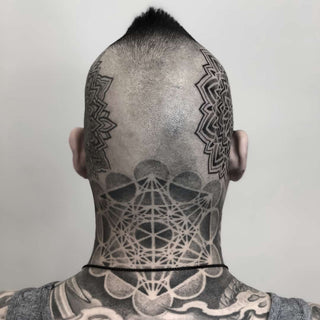This square photograph captures the back of a heavily tattooed white man's head and upper shoulders. He has a predominantly shaved head, except for a short black mohawk on top. The man is wearing a gray tank top and a thin black string around his neck. The tattoos covering his head and neck are intricately designed: On either side of his head are mandala-like tattoos, which incorporate pointy, wave-like patterns and flower petal shapes with shading that alternates between light and dark. Centrally located on the back of his neck, extending up to the base of his skull, is a complex geometric tattoo. This tattoo features black circles interconnected by white lines, forming a pattern that includes shapes like triangles, circles, and hexagons, with a prominent black circle at the center. The detailing creates a mesmerizing array of rays and lines that interlink the various elements, giving the entire tattoo an artistic, almost celestial appearance. While the tattoos continue onto his back, the image only captures the design up to his shoulders.